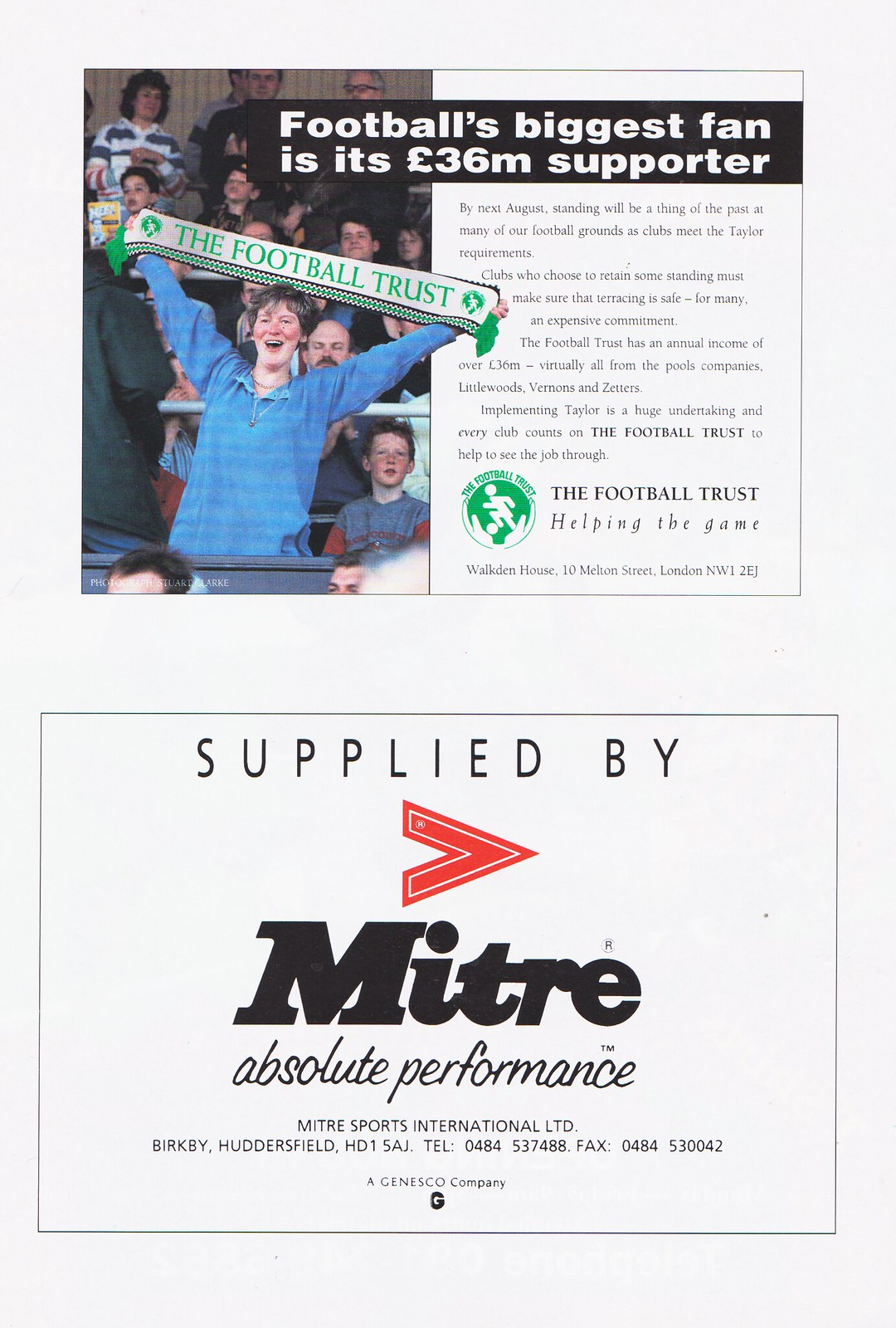The image consists of two vertically aligned advertisements, with the top ad focusing on football (soccer) and the bottom ad likely promoting performance tires. In the top ad, a young woman wearing a blue sweater is enthusiastically holding up a green scarf that reads "The Football Trust" in white letters against a black background. She stands amidst a crowd of fans, all seated and watching the game. A banner beside her proclaims, "Football's biggest fan is its 36 million pound supporter," highlighting a collective effort by companies to fund the sport. Below this, a smaller paragraph explains the creation of a 36 million euro fund by a conglomerate of companies to support football. The bottom ad, simpler in design, features black lettering on a white background with the message "Supplied by MITRE, Absolute Performance," and additional details about Mitre Sports International Limited, including their address and contact information. The ads suggest a juxtaposition of football support and sports equipment or performance products, and seem to be designed for print media such as a newspaper.